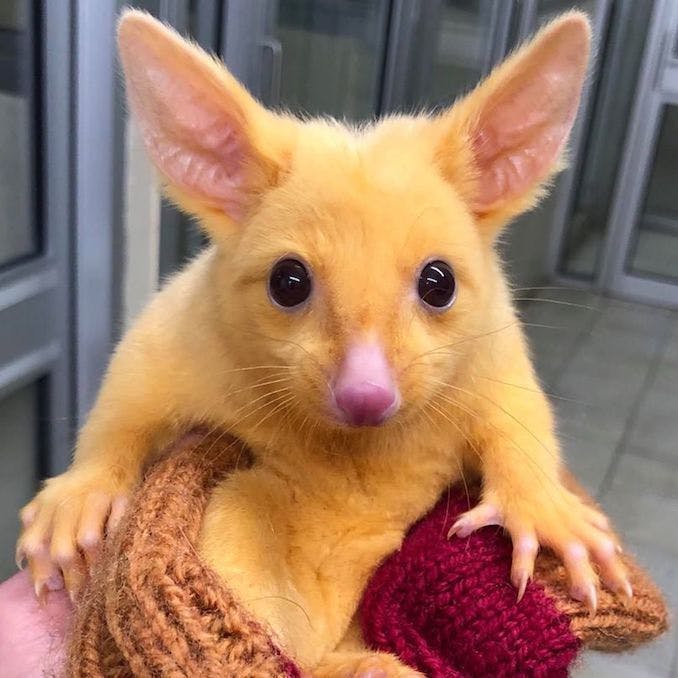The image features a vibrant golden-yellow rat with large pink ears standing straight up, beady black eyes, and a sizable pink nose. Its pinkish claws, dirty yellow nails, and long whiskers are clearly visible. The rat, with its fur suggesting an albino type or possibly dyed, is centrally positioned and staring directly at the camera, evoking a blank or surprised expression. It is partially wrapped in a maroon and brown knit scarf held by a person, whose arm is just visible at the lower left corner of the image. The setting is indoors with tile flooring and gray glass-panel doors in the background, suggesting the image might have been taken at night inside a building. The overall color palette of the image includes black, gray, white, yellow, pink, maroon, and light brown.